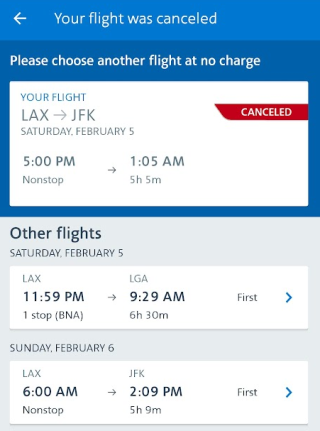This is a screenshot of a smartphone displaying a flight cancellation notification. The top banner is blue with a white left-facing arrow, accompanied by the text "Your flight was canceled." Below this, a message states, "Please choose another flight at no charge." 

In a white box beneath that, specific flight details are listed: 
- "Your flight: LAX → JFK, Saturday, February 5th, 5:00 PM non-stop, arrival at 1:05 AM, 5 hours and 5 minutes, canceled." 
- A red banner prominently displays "Canceled."

Beneath the cancellation notice, a gray box presents alternative flight options for the same date, Saturday, February 5th:
- The first option: "LAX, 11:59 PM → LGA, 9:29 AM," displaying the duration of 6 hours and 30 minutes with one stop (BNA). To the right of this option, the word "First" is displayed next to a blue right-facing arrow.
- The second option: "Sunday, February 6th, LAX, 6:00 AM non-stop → JFK, 2:09 PM," with a travel time of 5 hours and 9 minutes. Similar to the previous, it shows the word "First" followed by a blue right-facing arrow.

This webpage provides a notification of a flight cancellation along with options to select another flight at no additional charge.